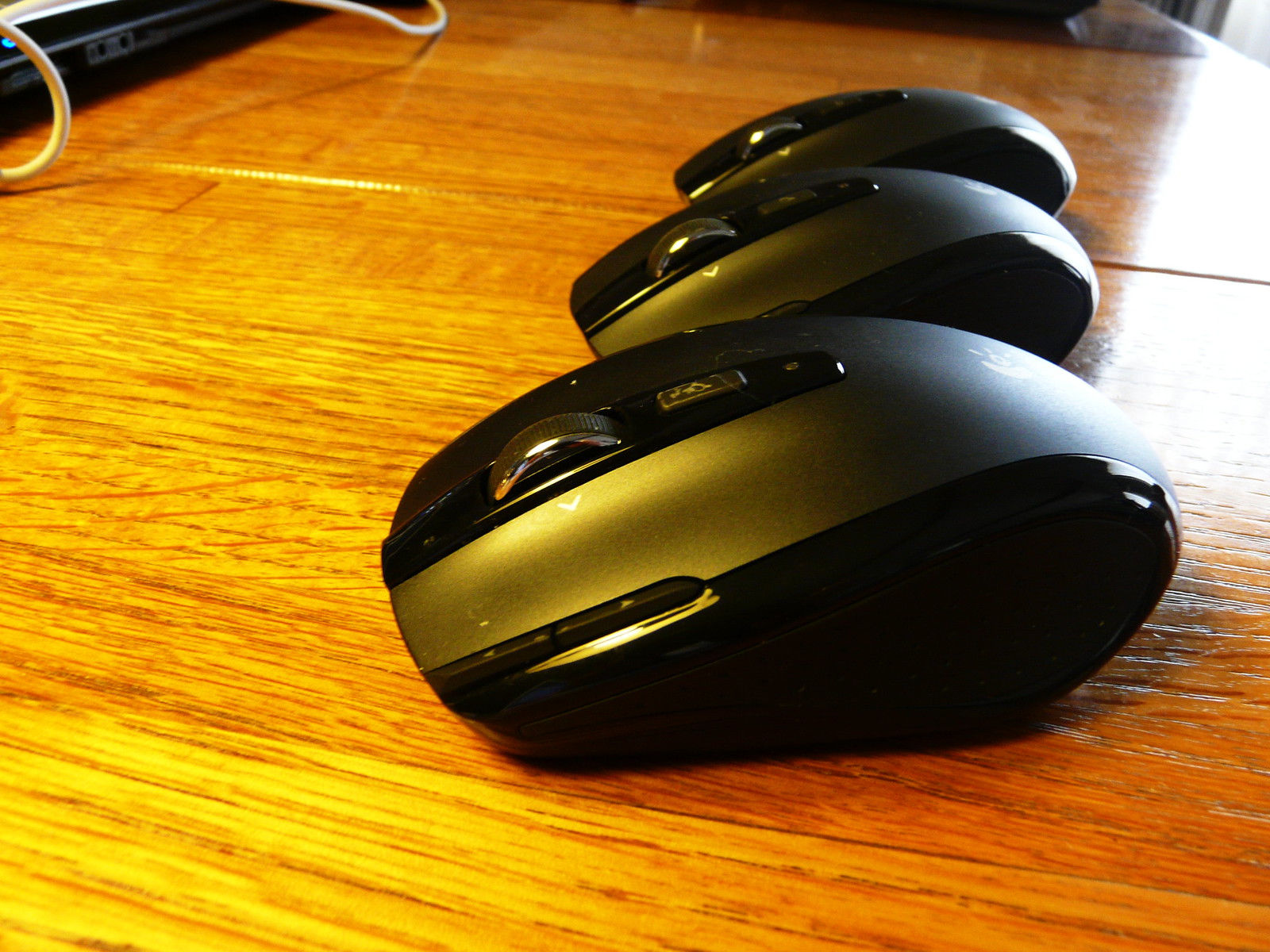In the image, we see three wireless computer mice placed on a medium-toned natural wood-finished table with horizontal planks. The mice, which are black with subtle gray detailing, are arranged with one in the foreground appearing slightly larger and the other two positioned to its side. The brown table is brightly lit, emphasizing its wooden texture. In the upper left corner, there is a hint of a computer monitor and two white electrical cords, suggesting a workspace setup.